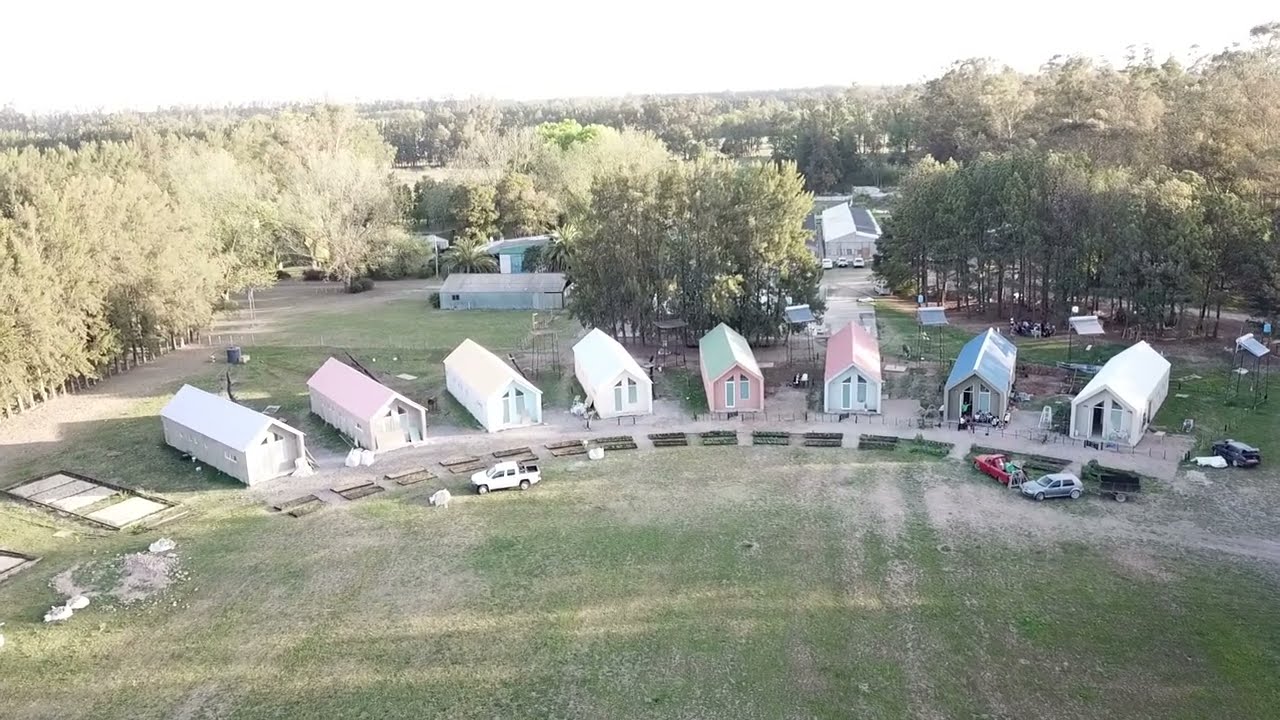The photograph captures a slightly overexposed daytime scene featuring a distinctive arrangement of approximately 8-10 small, shotgun-style houses or sheds. The buildings form an arch or half-circle, enclosing a central area of closely mowed green grass mixed with patches of white and brown dirt. Each structure is identical in form but uniquely painted, with varying colors such as white, green, red, and features roofs in shades of white, pink, blue, red, and green. Several cars are parked sporadically on the grass in front of the houses. Behind the row of buildings, tall trees dominate the background, with some additional homes or commercial buildings nestled among them, some appearing white and light green tin in color. The sky at the top of the photograph is washed out due to overexposure, blending into the treeline.